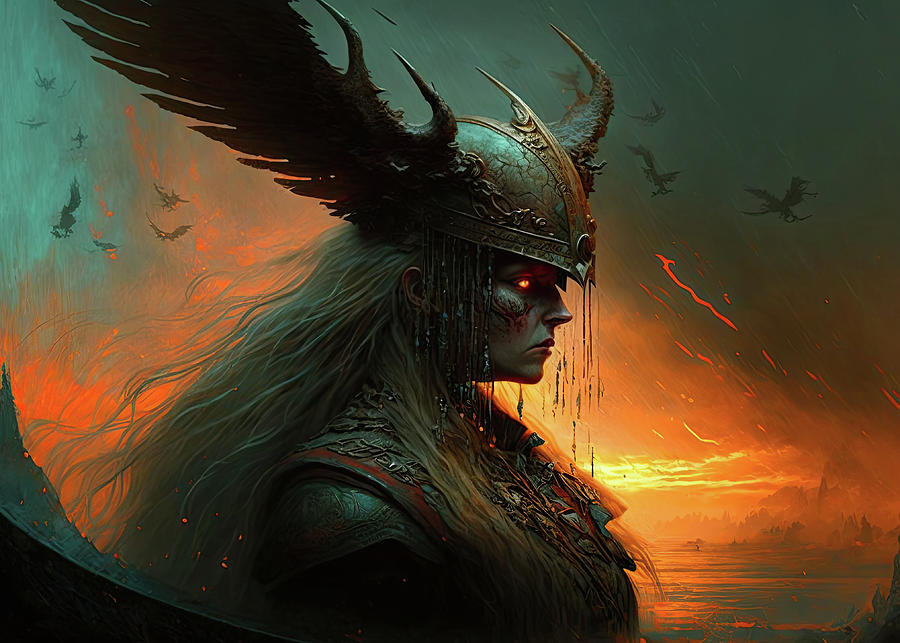The rectangular digital painting depicts a fantasy scene reminiscent of a video game or a graphic novel. It features a female warrior in profile, facing to the right. She has long, flowing white or blonde hair and dark, grayish skin, likely an artistic choice. Her eyes are glowing a striking red or orange. She is adorned in elaborate, heavy armor with intricate designs, and wears a unique helmet. The helmet has sharp spikes, and bony, wing-like structures protruding from the sides, adding to her fierce appearance.

Behind the warrior, the sky transitions from a vivid orange in the center to a deep blue at the top left, giving an impression of an apocalyptic setting. There are flying creatures, possibly bats or dragons, scattered across the sky. The right side of the image is engulfed in a striking gray tone with red flashes, contributing to the sense of turmoil. The background also suggests the presence of water and hints at a distant battle or war scene. Overall, the image is richly detailed and conveys a dramatic, fantasy atmosphere.